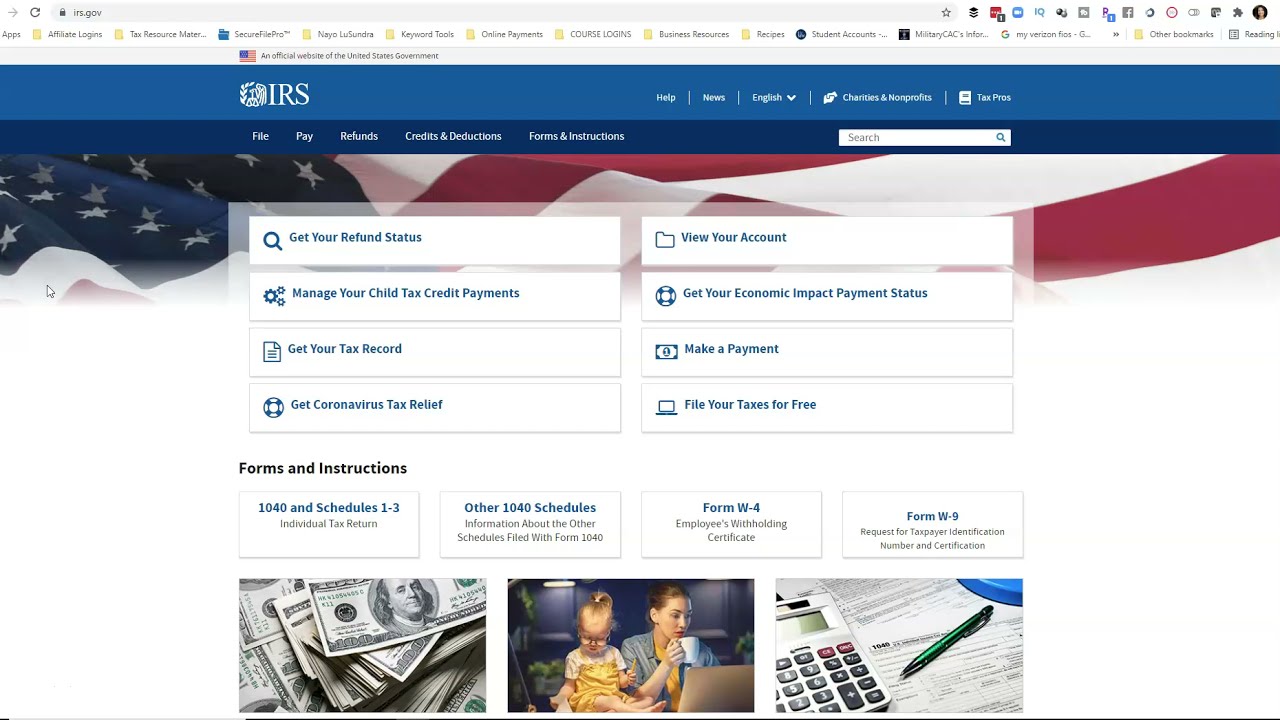The image depicts the "My IRS" portal interface, designed for various tax-related activities. The top of the webpage features a blue bar with the IRS logo prominently displayed. Below this, a deeper blue navigation bar offers five category selections: File, Pay, Refunds, Credits & Deductions, Forms & Instructions, and a search box situated on the right.

An American flag image is placed just below the dark blue navigation bar, followed by eight interactive boxes on a white background with blue text. These boxes offer key services such as checking your refund status, making a payment, obtaining your tax record, and filing your taxes for free.

Under these, there's a single row of four white boxes with titles and descriptions, each related to essential tax forms and instructions. The first box on the left is labeled "1040 and Schedules 1-3, Individual Tax Return." The second box highlights "Other 1040 Schedules." The third box is designated for "Form W-4," and the final box focuses on "Form W-9."

At the bottom of the page, three illustrative images are displayed. On the left, there is a photograph of a stack of money. The center image shows a young child sitting on a table next to her mother, who has a cup of coffee and an open laptop. The third image depicts tax forms accompanied by a calculator and a pen, lying on top of the forms on a table.